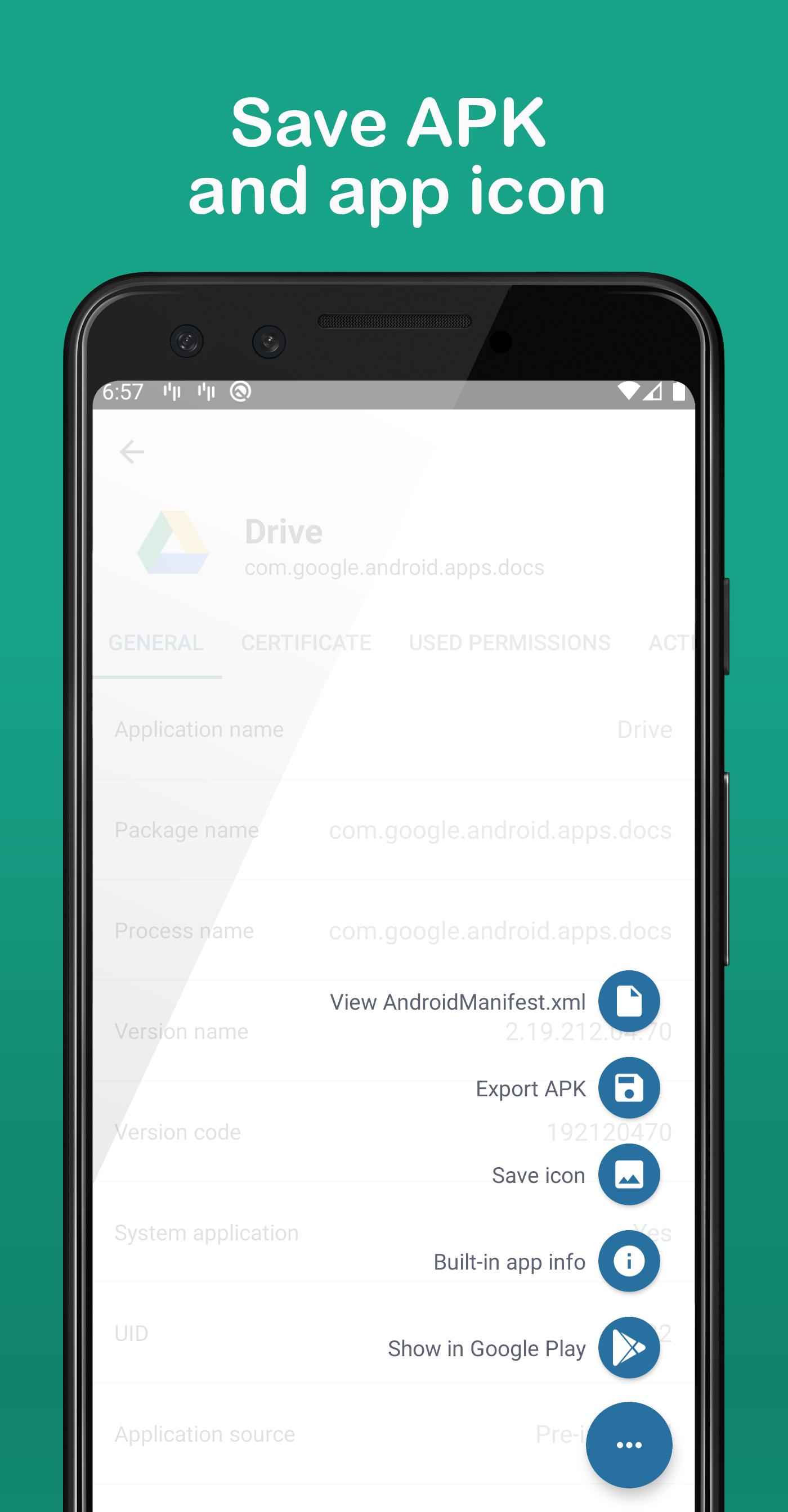The screenshot depicts a cell phone interface with a green background. The focal point of the image is the outlined shape of a cell phone screen. At the top section, the screen displays the word "SAVE APK" in bold, uppercase letters, accompanied by the text "App Icon" on the next line.

In the upper-left corner, standard notification icons are faintly visible along with the time, which is displayed as 6:57. The upper-right corner also features standard icons typically seen on a cell phone display.

Beneath this, the faint outlines of app icons for Chrome and Drive can be discerned, although they appear muted due to an overlay menu. The overlay menu prominently features several actionable items in descending order, each with a corresponding icon on the right. The menu options listed are: 

1. View androidmanifest.e.xml
2. Export APK
3. Save Icon
4. Built-in App Info
5. Show in Google Play

Each option is accompanied by a button icon, suggesting further interaction capabilities. 

The detailed design and layout suggest the image may be from a software or app development environment, where users can perform various tasks related to APK file handling and application management directly from the menu interface.